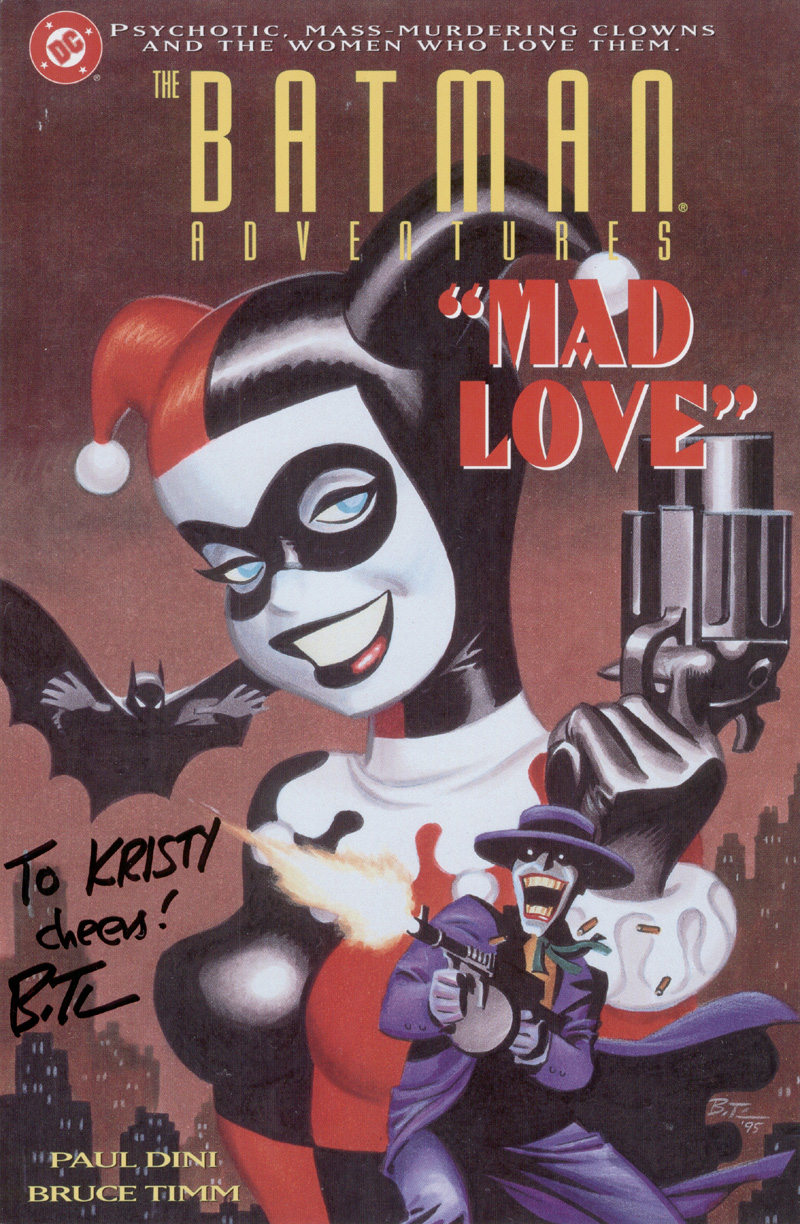The image is an autographed cover illustration for a DC comic or graphic novel titled "The Batman Adventures: Mad Love." Prominently featured in the center is Harley Quinn in her iconic red and black jester costume, holding a short-barreled revolver in her left hand. To her left, Batman is depicted flying forward, seemingly in motion to catch her. At the bottom right corner, the Joker, wearing his recognizable purple suit and a short-brimmed hat, is shown with a wide grin while firing a machine gun. The top of the image bears the text "Psychotic Mass Murdering Clowns and the Women Who Love Them." The DC logo is placed at the top left, consisting of white text on a red ring background. Below the title, "The Batman Adventures" is written in yellow, with "Mad Love" in red quotation marks. At the bottom left, the creators' names, Paul Dini and Bruce Timm, are displayed. Additionally, there is a personal inscription in black Sharpie reading, "To Christie, Cheers! BIT…"